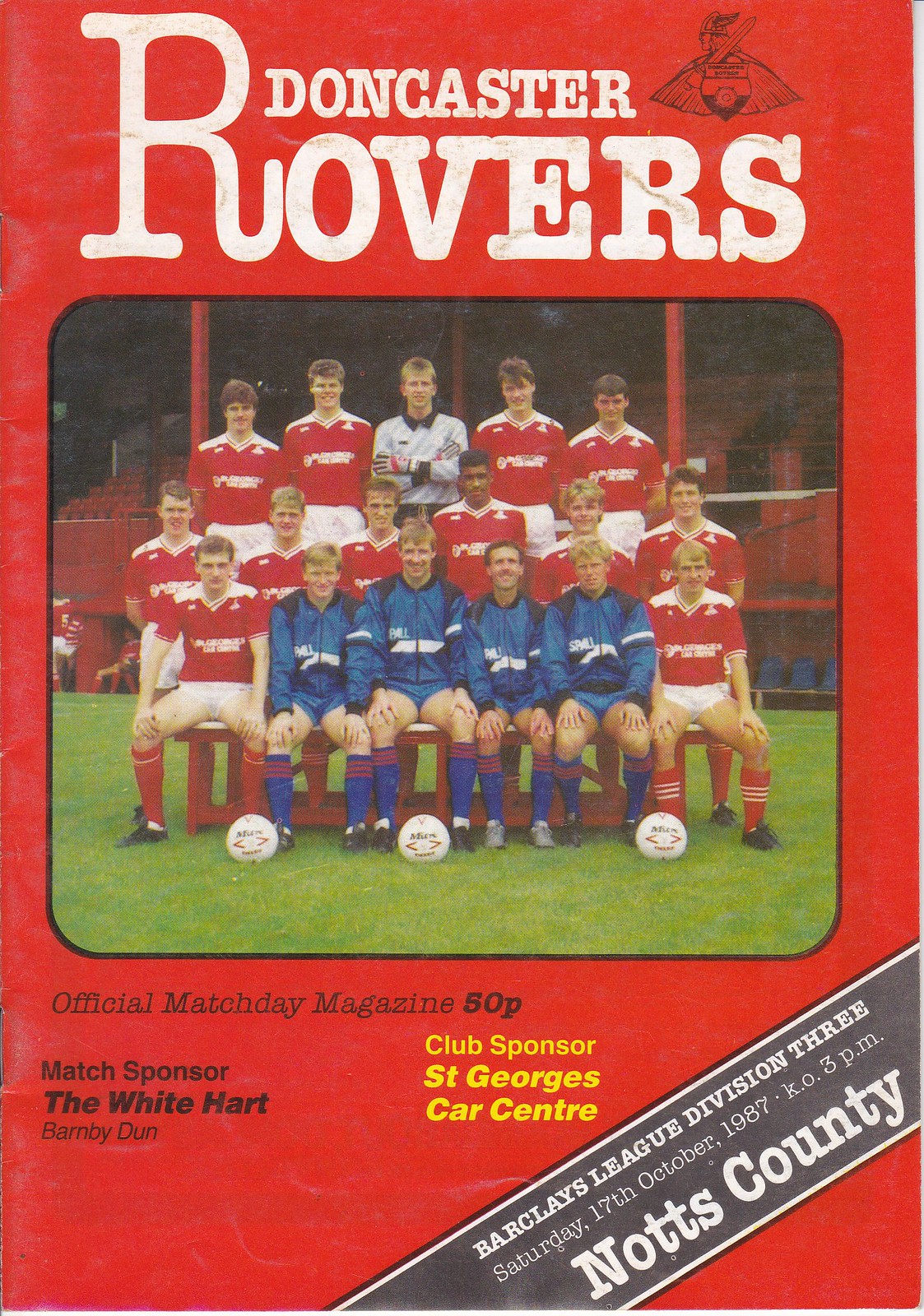The cover of the Doncaster Rovers official match day magazine, priced at 50 pence, is set against a striking red background. The focal point of the cover is a color photograph of the team, framed by a thin black border. Seventeen players are arranged in three rows – with the front row seated, the middle row standing, and the back row higher up, creating a pyramid-like structure. Four players in the front row wear blue uniforms, while the others predominantly wear red jerseys with white shorts and red socks, except for one player in the back row who is clad in a white uniform. Three soccer balls are placed in front of the team. The photo is taken on a green soccer field with empty bleachers in the background. The top of the cover features bold white text stating "Doncaster Rovers," and the bottom reads, "Official Match Day Magazine 50p. Match sponsor: The White Heart Barnby Dunn. Club sponsor: St. George Cars. Barclays League Division 3, Saturday 17th October 1987, Kickoff 3 p.m., versus Notts County."